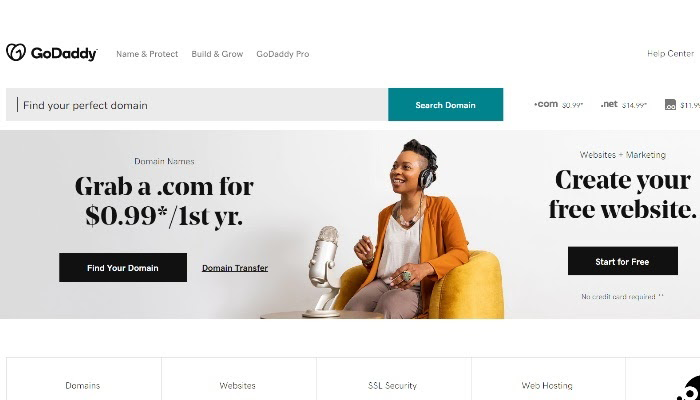Here's a polished and detailed caption for the image:

---

This screenshot showcases the GoDaddy web page. At the topmost section, the header features the GoDaddy logo on the left, which displays a heart-like symbol, followed by the name 'GoDaddy' in bold text. Adjacent to the logo are three navigational categories: "Name & Project," "Build & Grow," and "GoDaddy Pro." Towards the far right of the header, there's a link to the Help Center.

Beneath the header, a prominent search bar invites users to "Find Your Perfect Domain." Attached to this bar is a teal-colored button labeled "Search Domain." To the right of the search bar are domain extensions and their respective prices: .com and .net, followed by another box displaying a different price.

Below this section, a hero image with a gray background captures attention. The image features a woman relaxing in a yellow recliner, wearing headphones, and with a speaker placed in front of her. To the left of the image, text promotes "GrabAid.com for 99 cents first year" along with the callout "Find Your Domain." On the right side of the image, there's a promotion for "Create Your Free Website" with a button below it that invites users to "Start for Free."

At the bottom of the screenshot, a series of white boxes display various categories: Domain, Website, SSL Security, Web Hosting, and another partially visible category, hinting at additional options available off-screen.

---